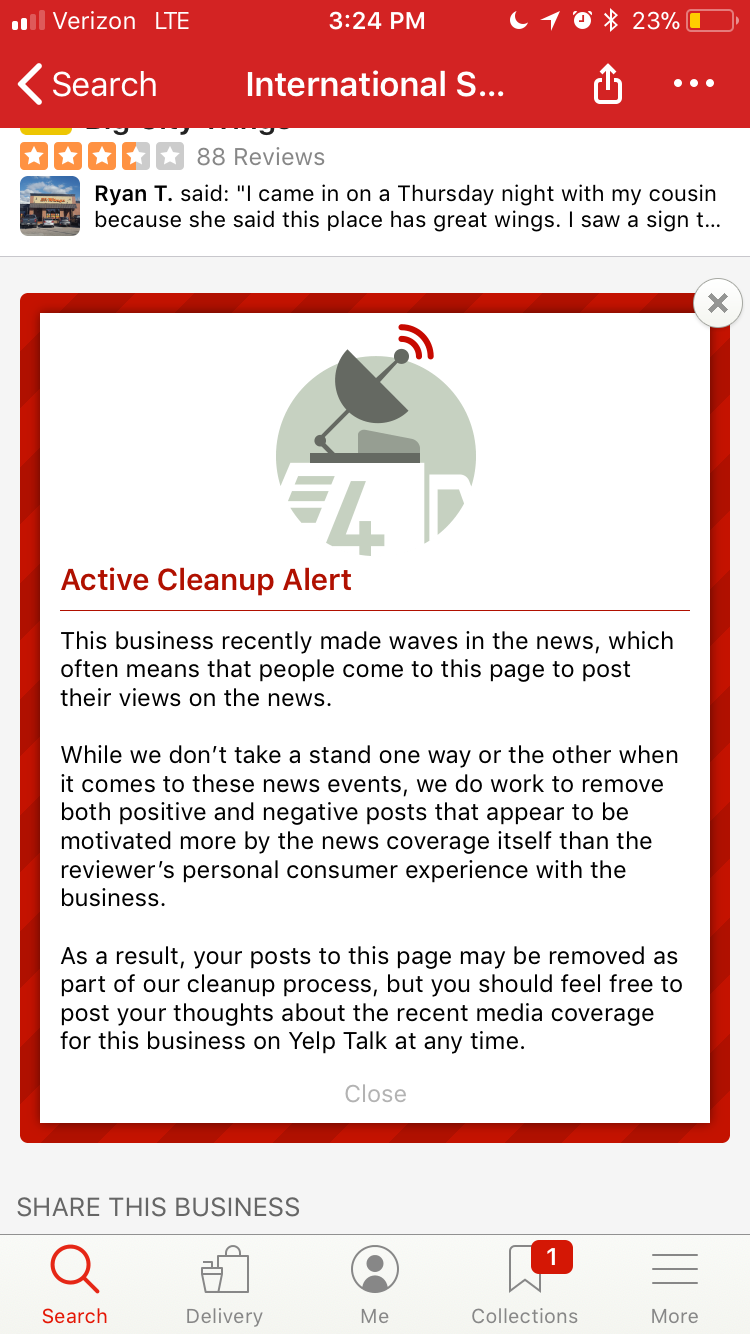The image showcases a screenshot taken from a cell phone. 

In the upper left corner, the phone interface shows a red signal strength indicator with cell phone bars, indicating the signal for Verizon LTE. The time "3:24 p.m." is displayed in the middle of the status bar. On the upper right, there are various icons including a crescent moon (Do Not Disturb mode), an alarm clock, a Bluetooth symbol, and a battery icon showing 23% charge, marked in yellow.

Below the status bar, the interface indicates a search field with a left arrow, a text snippet starting with "International s..." and an upload icon depicted as a square with an arrow pointing upwards, followed by three dots. The background of this section is white.

Partially visible above this, there is text from a review by someone named Ryan T. It begins with “I came on a Thursday night with my cousin because she said this place has great wings I saw a sign T..." but the rest of the review is cut off. 

An alert pop-up with a thick red outline around it also appears on the screen. In the upper right corner of the alert is an 'X' for closing it. The alert text reads:

"Active Cleanup Alert
This business recently made waves in the news which often means that people come to this page to post their views on the news. While we don't take a stand one way or the other when it comes to these news events, we do work to remove both positive and negative posts that appear to be motivated more by the news coverage itself than the reviewers' personal consumer experience with the business. As a result, your post to this page may be removed as part of our cleanup process. But you should feel free to post your thoughts about the recent media coverage for this business on Yelp Talk at any time."

Based on the pop-up alert, it can be inferred that this screenshot is from the Yelp app.